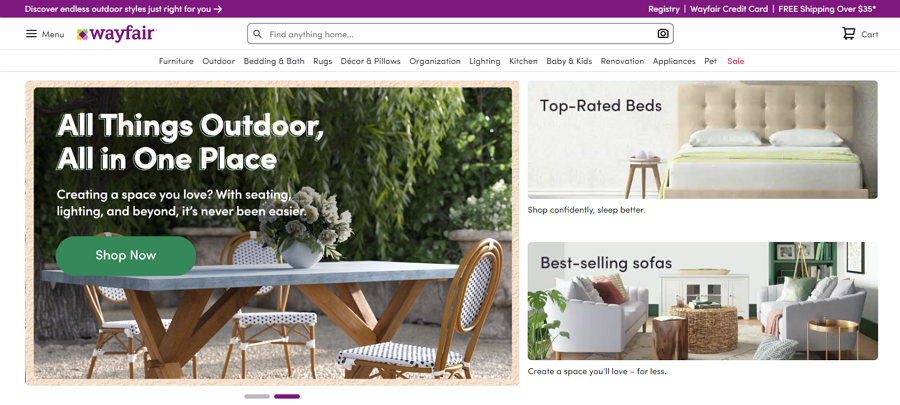Screenshot of the Wayfair homepage. The top navigation bar is purple and quite dense with information. At the very top, there is a search bar. Below this bar, various subsections are displayed, including "Furniture," "Outdoor," "Bedding & Bath," among others.

The homepage highlights three main promotional links with professional images corresponding to each:
1. "All Things Outdoor, All in One Place. Shop Now."
2. "Top Rated Beds."
3. "Best Selling Sofas."

The layout is a wide cropped shot of the site. Additional features include a registry button and an advertisement for the Wayfair credit card. Free shipping is offered on orders over $35. A menu button is located at the top left corner, which reveals more options upon clicking. The overall design is professional yet typical for an online retail site, ensuring usability but not particularly distinctive.